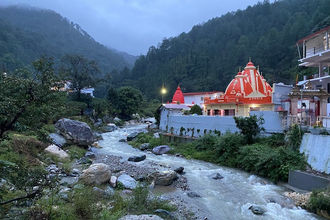The photograph captures a tranquil scene of a small town nestled in a mountainous region, likely in a foreign country. The background is dominated by majestic hills and mountains adorned with lush green trees, fading into a cloudy or foggy sky. At the center and to the right of the image, there is a multi-story building, possibly a residence, that stands near a distinctive large red or orange pyramid-shaped structure, which could be part of a circus or another unique landmark. A small creek meanders through the scene, framed by wetlands, rocks, and patches of grass on its left side. Just next to the buildings, there is a white, solid fence made of concrete, marking the area. There are also two domes with red accents: one larger dome-topped building and a smaller adjacent dome. The picture evokes a sense of serene beauty with its combination of natural elements and the quaint architecture of the town.